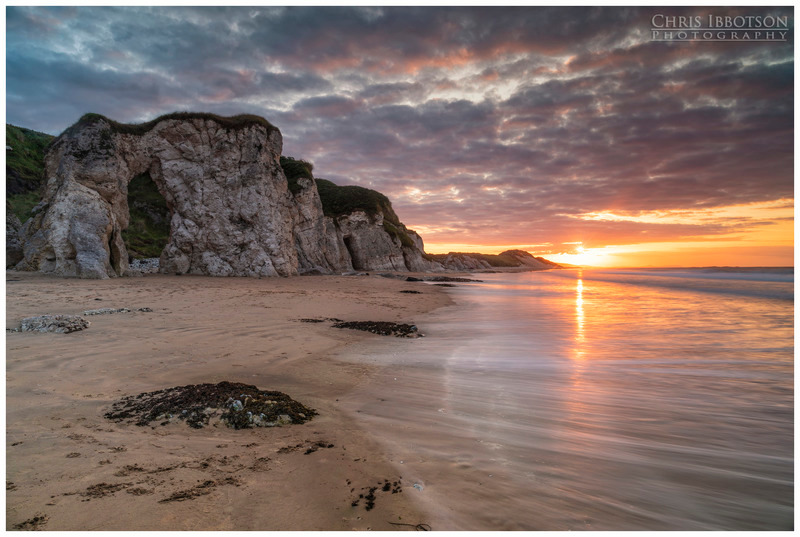A stunning color photograph captures a tranquil beach scene at sunset. The sun, a glowing orange orb, is near the horizon slightly to the right, casting its golden reflection on the calm, foamy waves of the sea. Dark silhouetted clouds, tinged with purples and blues, provide a dramatic sky, while the beach below extends from the middle of the frame toward both the left and right edges. Toward the left stands a bluff, about two stories tall, with some grassy tufts on top, and a notable rock formation featuring a hole. The dark, fine sand of the beach, sprinkled with a few black rocks and some seaweed, shows no signs of human presence, enhancing the serene and untouched beauty of the landscape. The photograph, signed in the upper right corner by Chris Ibbotson Photography, captures the essence of a peaceful coastline bathed in the enchanting hues of sunset.